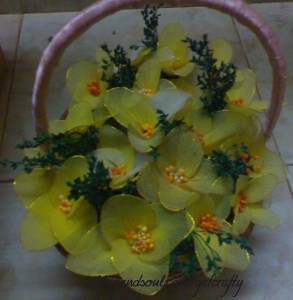The photograph depicts a slightly dark and low-quality image of a flower arrangement in a pink basket, reminiscent of an Easter display. The basket features a long, arching pink handle that curves above the cluster of flowers. The flowers, which are a blend of mustard green with bright yellow edges, have four oval-shaped petals tapering to a point, arranged in a cross pattern. The centers of these synthetic flowers contain spherical, multicolored beads, predominantly orange, adding a vivid focal point to the arrangement. Among the flowers, small green sprouts resembling pine needles extend outward, enhancing the bouquet's ornate design. The leaves appear to be synthetic and somewhat transparent, further indicating the artificial nature of the bouquet. At the bottom of the photograph, there is faint, unreadable text that might denote the creator or photographer of the bouquet.